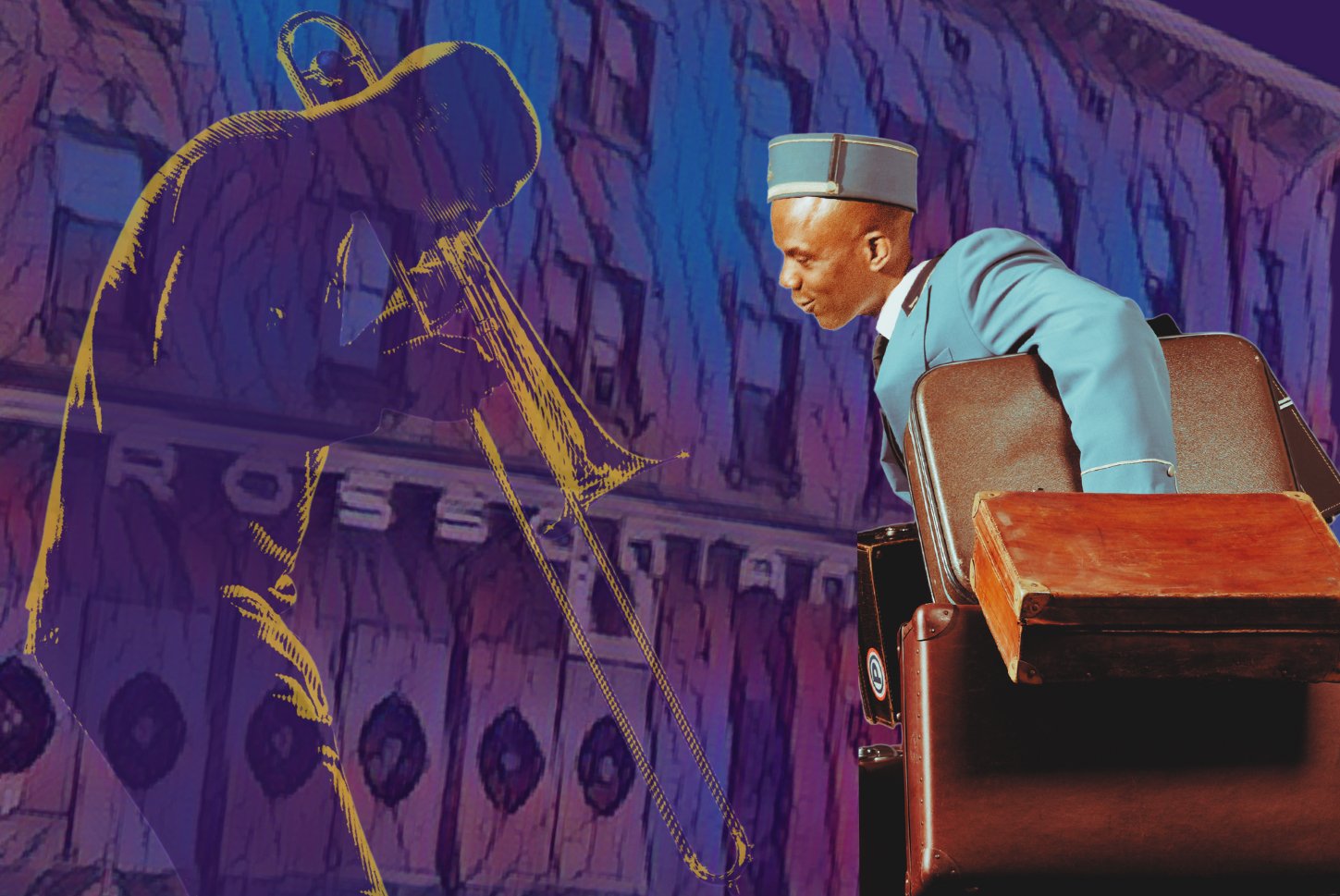This highly detailed and well-executed illustration captures a poignant moment outside a venue or place named "Rossinarium." On the right side, there is a realistic portrayal of a black man, dressed as a bellhop in a light teal uniform and hat, carrying multiple suitcases and bags. His posture is attentive, and he has a smirky smile on his face as he looks towards the left side of the image. On the left, there's a hand-drawn, slightly transparent and yellow-tinted depiction of another black man, bent over and deeply engrossed in playing a trombone, with the instrument pointed towards the ground. The trombone player appears almost ghost-like, rendered in a stencil style that contrasts with the more lifelike depiction of the bellhop. The background features dark purple and blue tones that suggest the façade of a building, creating a rich, atmospheric backdrop for the characters. The illustration seamlessly blends different artistic styles to highlight the emotional and observational dynamic between the two characters, with the bellhop seemingly lost in the music or memories evoked by the trombone player's soulful performance.